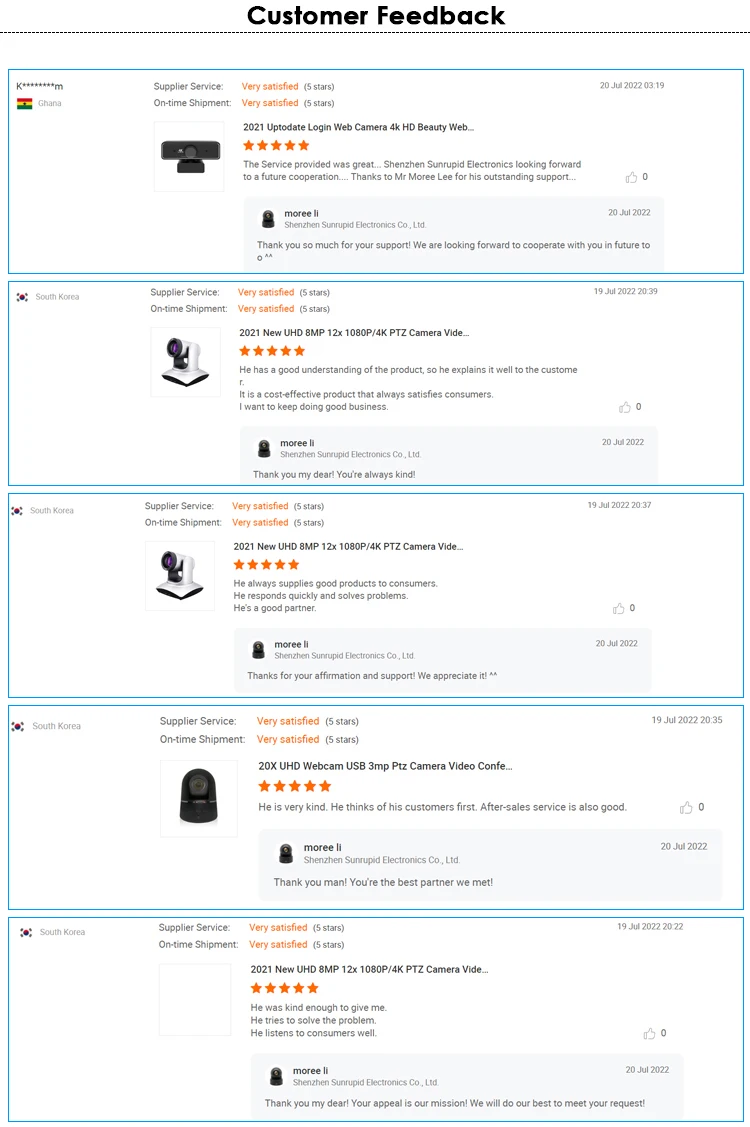"Introducing the latest in webcam technology for 2021: a state-of-the-art PTZ camera featuring an ultra-high definition (UHD) resolution of 4K. With an 8-megapixel sensor, this cutting-edge device offers a 12x optical zoom and an expansive wide-angle view. Perfect for video conferencing, the camera supports full HD 1080p streaming and is equipped with USB 3.0 connectivity for seamless integration. This versatile webcam is lauded for its exceptional performance and reliability, earning consistent 5-star reviews from users. Available in black and white, the camera is backed by supplier services from both China and South Korea, ensuring top-notch quality and customer support. First released on July 20th, 2019, this model continues to be a popular choice through 2022, solidifying its reputation in the market."